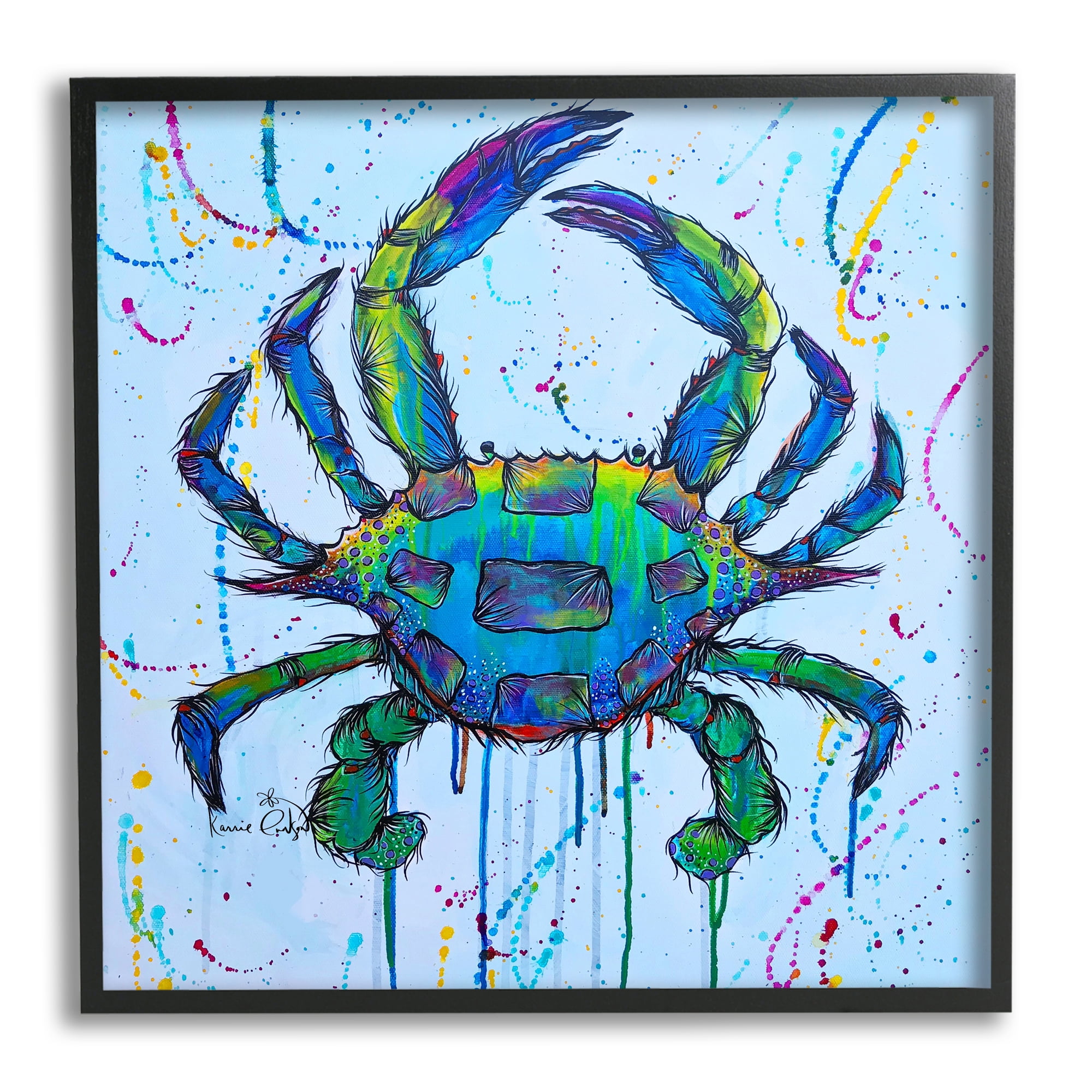This is a color photograph capturing a framed watercolor painting of a crab, displayed against a white wall. The painting, enclosed in a minimalistic black wooden frame, features a vibrant and multicolored crab viewed from above, with its head and eyes positioned at the top. The crab's body and claws predominantly exhibit shades of blue and green, accented by streaks of purple, splashes of red and orange, and occasional highlights of yellow. The crab is also covered with black hair extending from its surfaces. Its eyes, depicted as small black circles, are prominently visible at the top. The background of the painting is a light blue, interspersed with vibrant paint drips and splatters of yellow, purple, and green, creating a dynamic backdrop that integrates with the dripping ink effect from the crab. The artwork is signed by the artist between the lower two legs on the left side, although the signature is somewhat indecipherable. This colorful, detailed painting evokes the sensation of viewing a crab through a thermal camera, with its vivid, rainbow-like coloration.